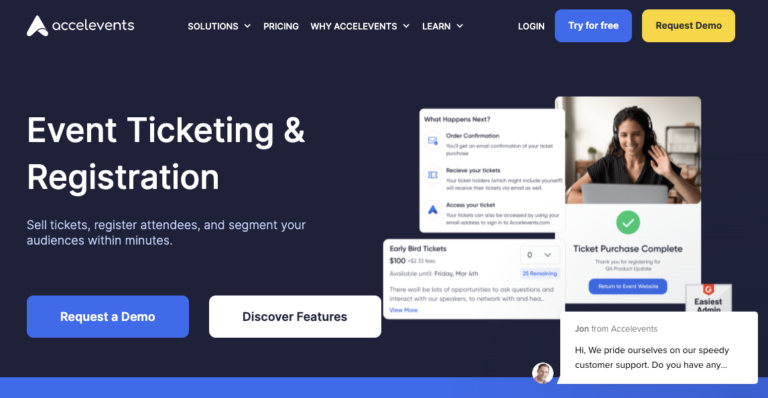This screenshot from a website features a sleek, dark-themed background with the Excel Events logo prominently displayed in the top left corner. A navigation menu follows, listing options such as Solutions, Pricing, Why Excel Events, and Learn. On the right-hand side of the header, there are three interactive buttons: Login, Try for Free, and Request Demo.

Dominating the left side of the main section is a compelling headline: "Event Ticketing and Registration," followed by a brief description: "Sell Tickets, Register Attendees, and Segment Your Audiences Within Minutes."

To the right, a collage of images showcases various facets of the platform. The central image features a woman working on a laptop. Surrounding this centerpiece are smaller, context-relevant visuals. To the left, there is text associated with ordering, possibly highlighting the ticket purchasing process. Below it, "Early Bird Tickets" is mentioned along with additional related text. On the right, a notification reads "Ticket Purchase Complete" next to a prominent green check mark, indicating a successful transaction.

In the bottom-right corner, a chat box demonstration is visible, showcasing customer support. A message from a representative named John states, "Hi, we pride ourselves on our speedy customer support. Do you have any...," emphasizing the company's commitment to customer service.